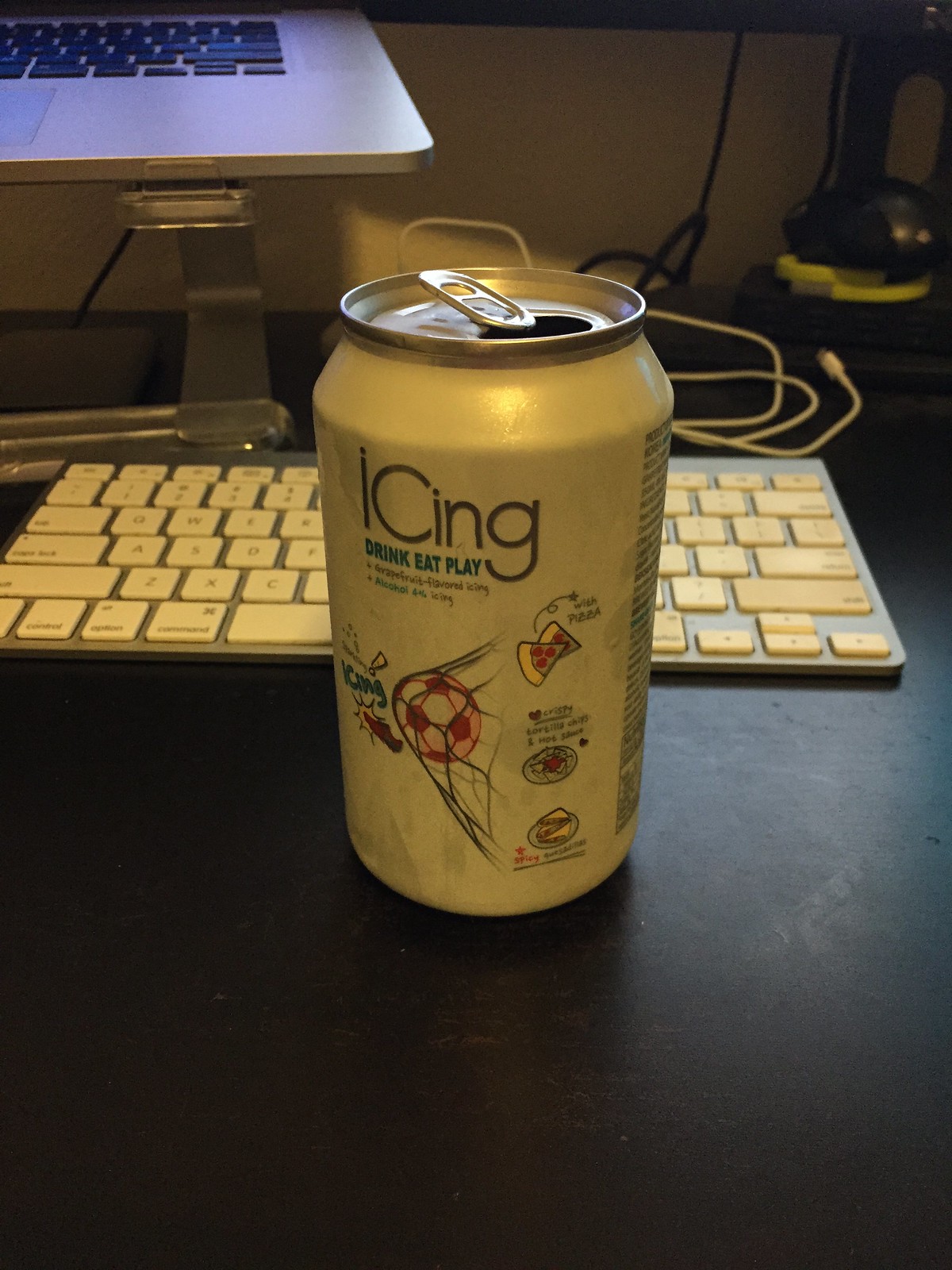This image showcases a white aluminum beverage can placed on a black desk or surface. The can prominently features the text "Icing" at the top, followed by the slogan "Drink, eat, play." The can is decorated with small illustrations including a soccer ball, a pizza slice, and a sandwich cut into triangles. The beverage can, which is open and lightly soaked, is positioned in front of a computer keyboard with white keys and a silver frame. Further behind, there is a clear plastic laptop stand supporting a silver laptop with black keys partially visible in the top left corner of the image. All the elements suggest this is a workspace setting.